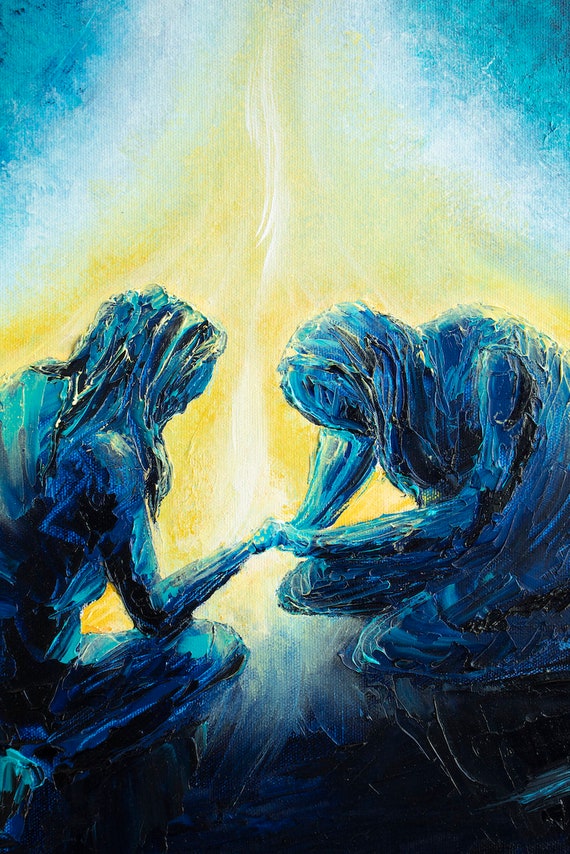This detailed painting features two blue-toned figures whose individual features are indistinct but clearly represent two people in an emotionally charged moment. Set against a striking backdrop split into a dark, almost black background with a prominent yellow central area that evokes the image of a fierce flame or radiant light, the painting exudes an aura of hope and energy. The figures dominate most of the canvas, occupying approximately three-fourths of the frame both horizontally and vertically. These two silhouettes, infused with vibrant shades of turquoise, blue, white, and yellow, appear to be kneeling or crouching, with their right arms extended towards each other, hands touching or holding. This gesture implies a deep connection, perhaps offering comfort or support in a moment of crisis. Around them, the interplay of dark blues and yellows adds a dynamic and poignant sense of shading and depth, further enhancing the painting’s emotional resonance.